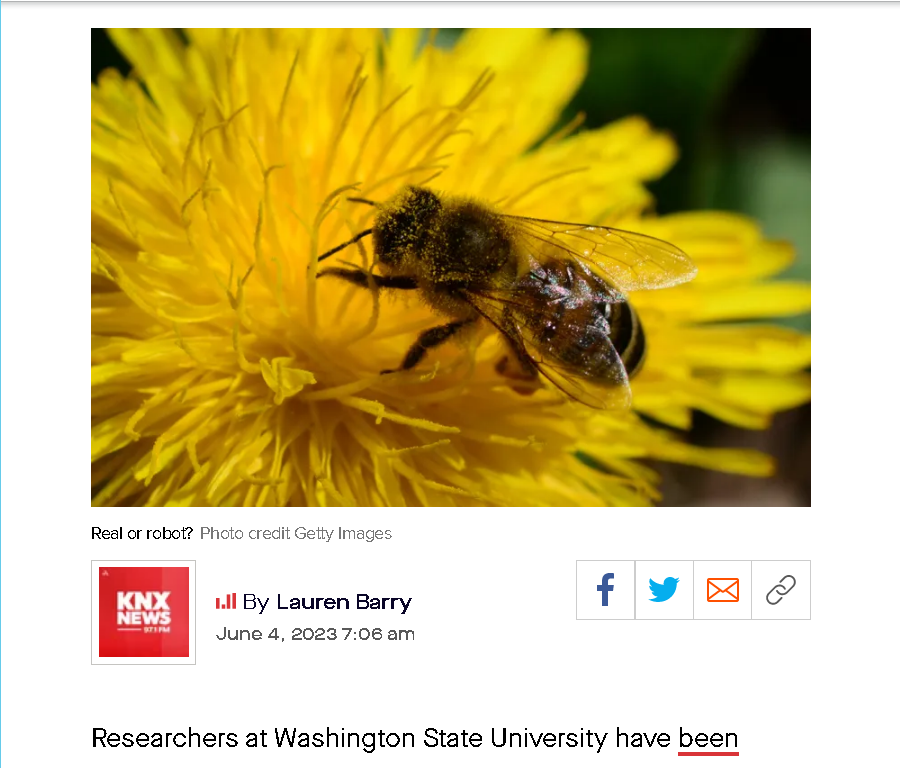In this detailed screenshot, a vibrant image takes center stage, capturing a bee delicately perched on the middle of a striking, bright yellow flower, which could be a dandelion or marigold. The flower's intricate petals fan outwards, with slender leaves visible underneath the blossom. Below the photo, a caption reads "Real or Robot," attributed to Getty Images. To the left, a prominent red box labeled "KNX News" can be seen.

Adjacent to the red box, the author's name, Lauren Barry, is displayed, followed by the date and time of the post. On the right side, four square icons for Facebook, Twitter, Email, and Link are presented, facilitating easy sharing of the article. Just beneath these elements, the beginning of an article is visible, with an introductory sentence about researchers at Washington State University, though the text "is" is conspicuously underlined in red, possibly indicating an editorial marker.

The page appears to be cropped, showing only the photo, author's name, source, and a fragment of the article text. A light gray bar spans the top of the screenshot, marking the crop's boundary, while a very thin blue vertical bar runs along the left edge, adding a subtle accent to the layout.